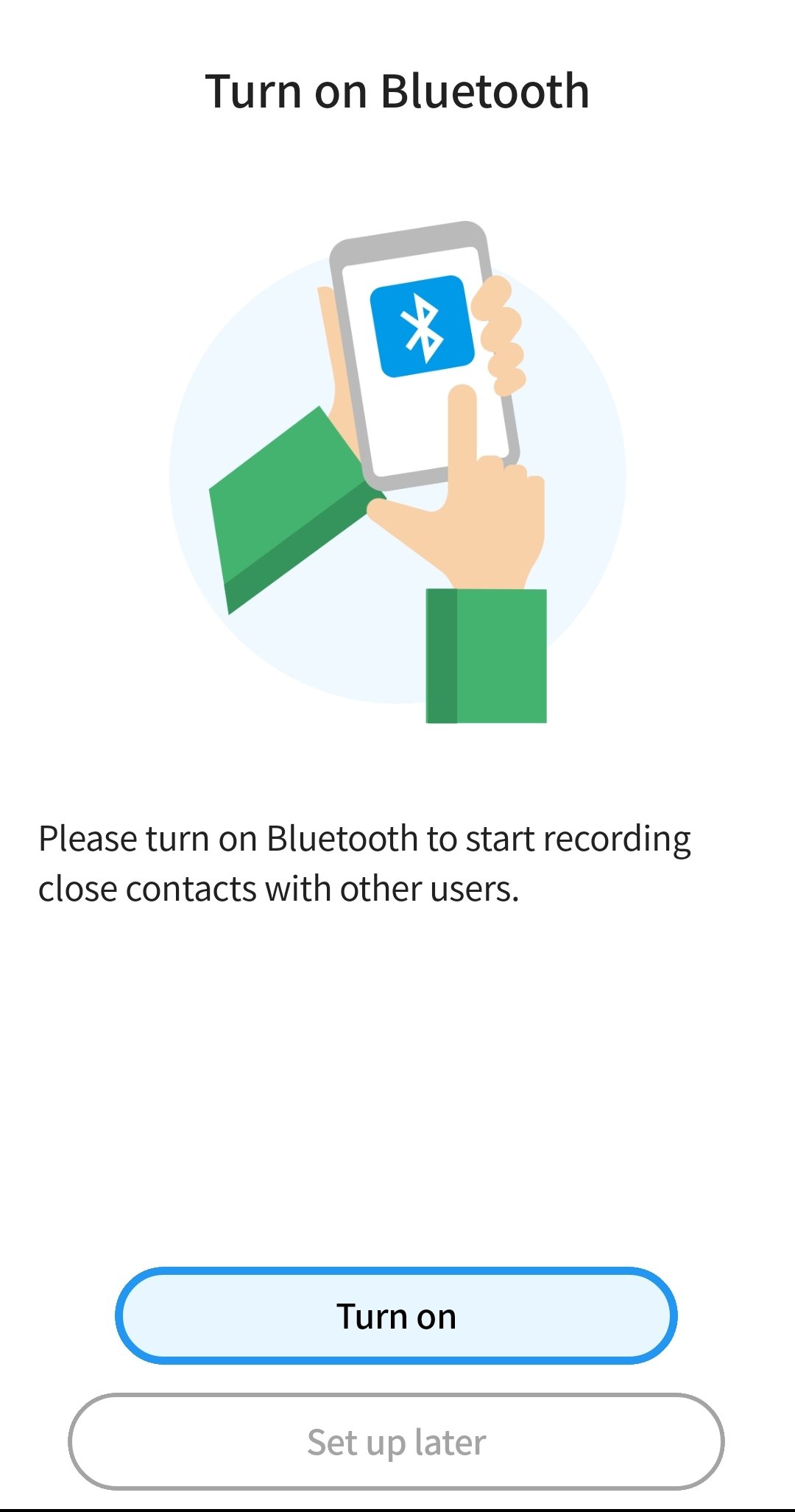Caption: The image is a screen capture from a mobile device showcasing a white background. Central to the image is a graphical illustration depicting a hand holding a mobile device while another hand points to the screen. The mobile device screen displays a Bluetooth icon in blue and white. At the very top of the image, in black text, the words "Turn on Bluetooth" are prominently displayed. Below this text, the illustrated hands interact with the device and the Bluetooth icon. The hands' sleeves are colored green. Further below, additional black text instructs, "Please turn on Bluetooth to start recording close contacts with other users." At the bottom of the screen, there are two rectangular buttons with curved edges. The first button is light blue with black text that reads, "Turn on." The second button, grey in color with black text, states, "Set up later."